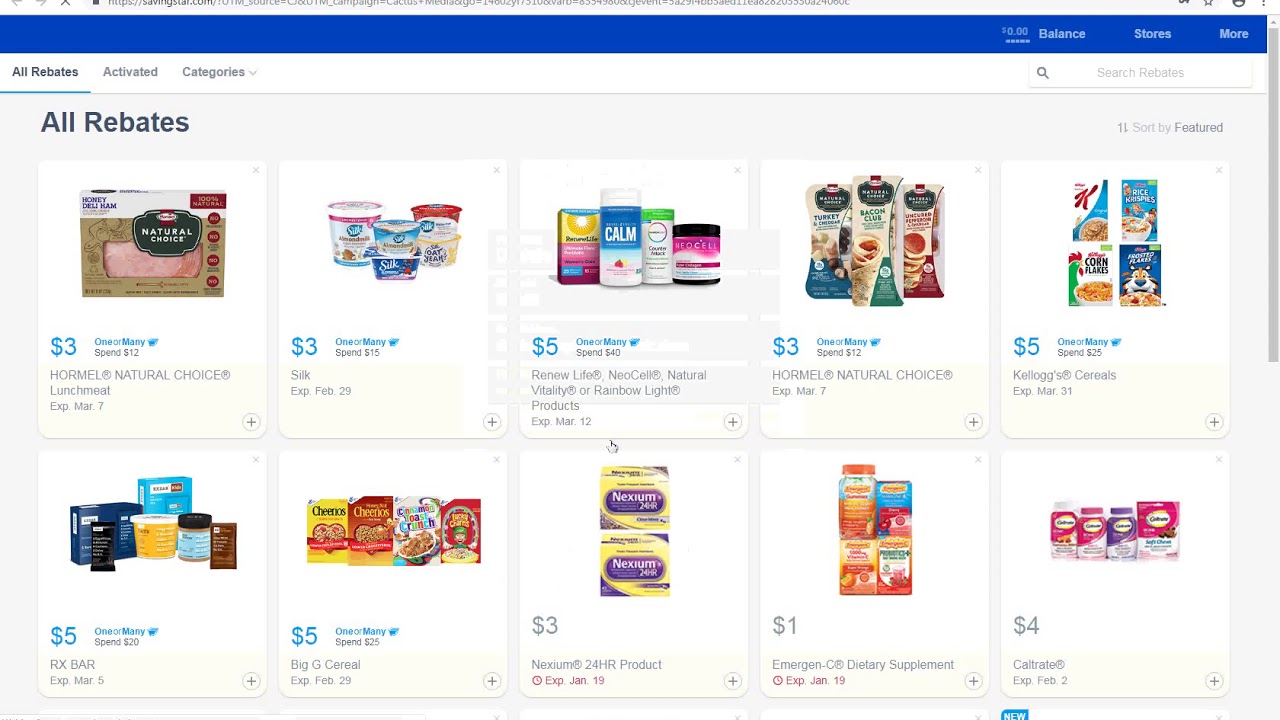The image appears to be a screenshot from the SavingStar website, which is identifiable by its URL visible at the top of the screen. The header features a blue border at the top and a white border on the right side, with navigational options labeled "Balance," "Stores," and "More." Below the header, the main interface starts with a white background and includes an option titled "or rebase," marked in a bold teal color, indicating user interaction. Following this, the text "aggregate categories" appears.

Beneath this initial section, the background transitions to light gray and displays the text "or rebates" in black. The content area is organized into two rows, each containing five product listings. 

In the first row:
1. **$3.00** - Hormel Natural Choice Lunch Meal, expires March 7th.
2. **$3.00** - Silk X, expires February 29th.
3. **$5.00** - Renew Life, NeoLife Natural Fertility, or Rainbow Light Products, expires March 12th.
4. **$3.00** - Hormel Natural Choice, expires March 7th.
5. **$5.00** - Kellogg's Cereals, expires March 31st.

In the second row:
1. **$5.00** - RX-BAR, expires March 5th.
2. **$5.00** - BG Cereal, expires February 29th.
3. **$3.00** - Nexium 24-hour product, expires January 19th. (Note that the dollar sign here is presented in gray, with the expiration date in red)
4. **$1.00** - Emergen-C Dietary Supplement, expires January 19th.
5. **$4.00** - Caltrate, expires February 2nd. (Here, the expiration date is shown in gray)

The product descriptions include the price in blue text and the product details in black, offering a clear visual distinction for users.